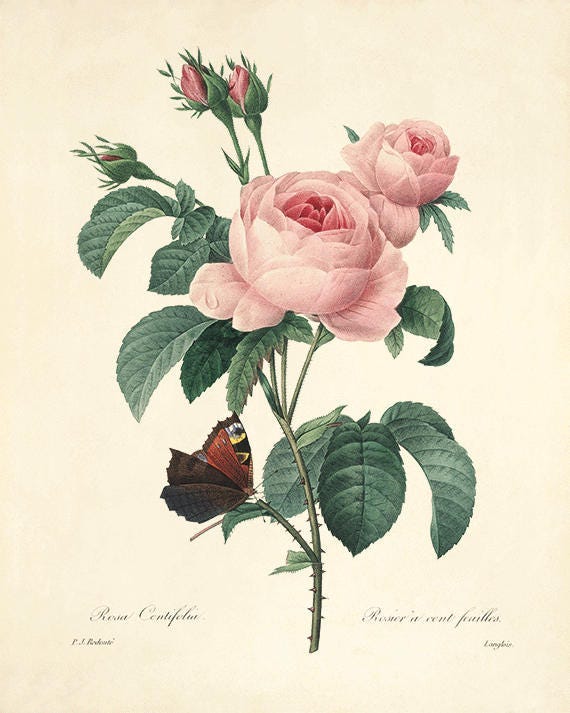The image is an antique-styled illustration of pink roses, likely created with colored pencils. At the top of the composition, there are three rose buds, slightly open, positioned above a prominent, fully bloomed pink rose in the center. To the right of this central rose, another more closed pink rose is visible. Dark green leaves and a thorny green stem provide a contrasting backdrop to the delicate petals. Along an offshoot of the main stem on the left, there is a brown moth adorned with white and black patterns. The illustration includes scripted writing in the bottom corners, though it is unreadable. The image, printed on off-white paper, features intricate details such as a bead of water on one petal of the central rose, and the inner petals displaying a deeper, almost burgundy hue.